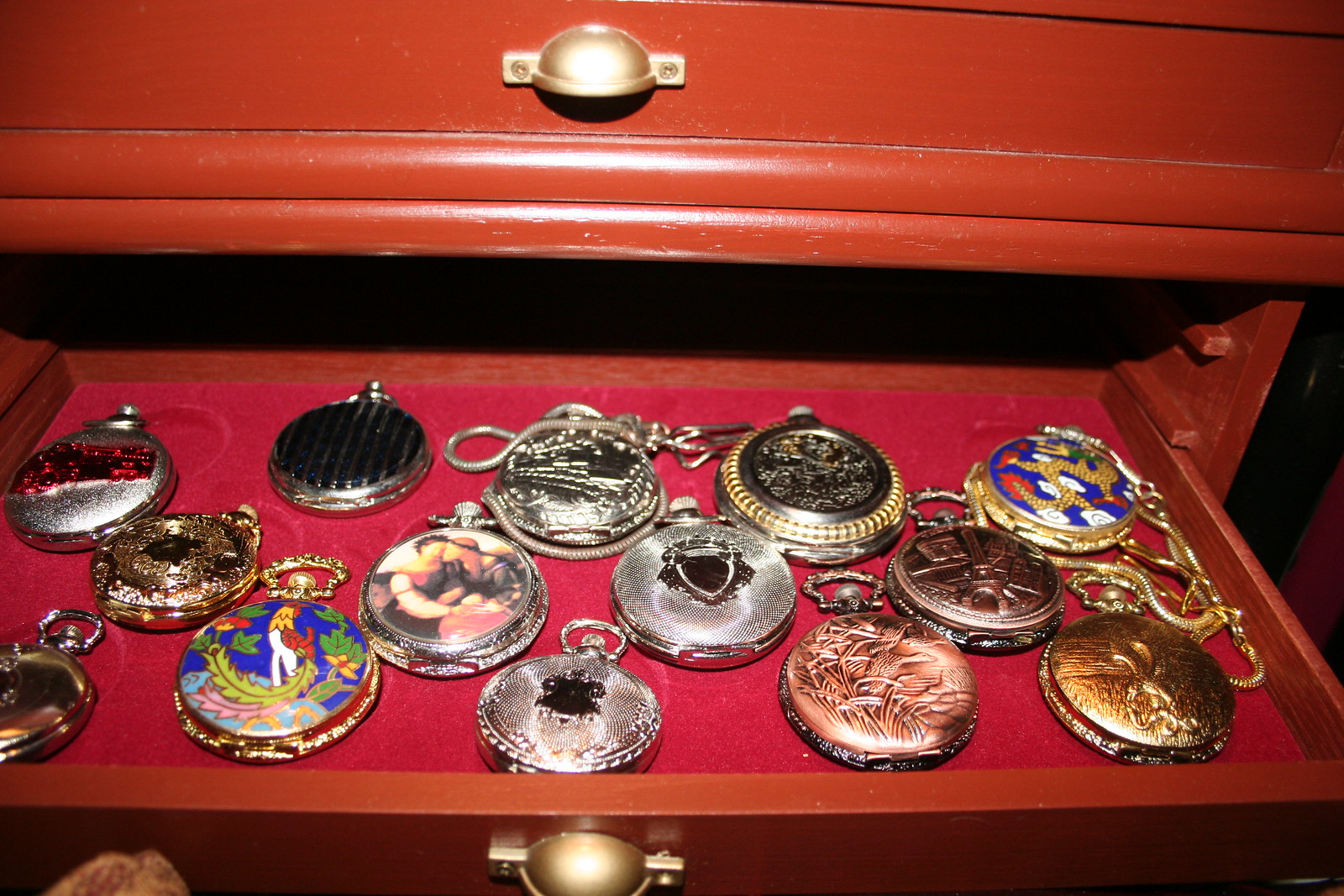This detailed photograph, taken indoors in landscape mode, showcases a collection of 14 pocket watches meticulously arranged inside an open drawer. The drawer, crafted from a bright orangish brown wood, features brass handles and has been pulled out to reveal a luxurious red velvet backdrop. These pocket watches are of various designs and colors, adding a captivating diversity to the display. Among them, there are three completely silver watches, a couple with rich gold finishes, and some boasting intricate enamel artwork. Notably, two of the watches feature vibrant, colorful designs, including bird motifs, and another displays a red element. Additionally, some watches have chains affixed to their loops, enhancing their display-ready presentation. The shallow drawer's foreground emphasizes the detailed craftsmanship of both the timepieces and the drawer, with the top half of the image focusing on the rest of the closed chest, complete with a yellow knob handle. The light hitting the surface of the watches highlights their polished exteriors, making them gleam against the rich, velvety red background.